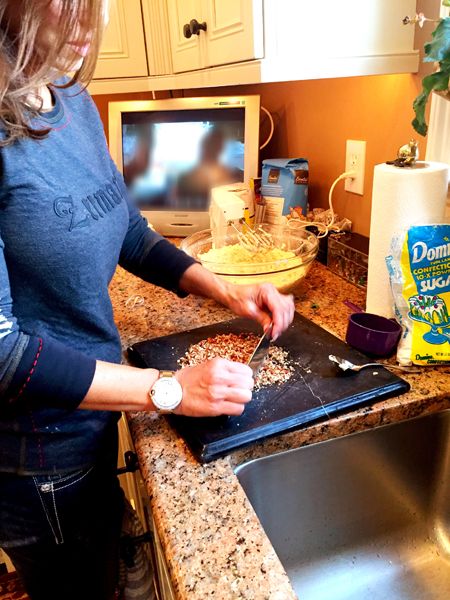A woman is meticulously preparing ingredients in her modern kitchen. Positioned under white cabinets, a computer screen is tucked away in the corner, potentially displaying a recipe or entertainment as she works. Below the cabinets, sleek marble or granite countertops gleam, housing an inset sink that remains unused for now. 

The woman wears a long-sleeved shirt with a partially visible inscription and pairs it with jeans. Her long hair cascades down her back, and she sports a prominent watch on her right wrist. At the moment, she is carefully chopping walnuts on a sturdy stone cutting board, holding the knife with both hands for precision.

Beside her, a paper towel rack stands next to a bag of Domino confectioner's sugar, while a glass mixing bowl, previously used for beating ingredients, awaits additional elements. The overall scene suggests she’s in the midst of creating a culinary delight, combining the chopped nuts into her mixture. The well-organized space and state-of-the-art equipment highlight an efficient and thoughtfully designed kitchen.